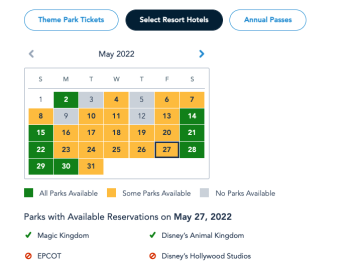This image is a cropped screenshot of the Disney World Park calendar, featuring a white background. The top section includes three navigation options: "Theme Park Tickets," "Select Resort Hotels," and "Annual Passes." The "Select Resort Hotels" option is selected, indicated by a dark blue bubble.

Beneath these options, a calendar is displayed on the left. At the top of the calendar, "May 2022" is printed in small blue letters, flanked by left and right arrows to navigate through different months. The calendar grid lists the days of the week at the top, followed by their corresponding dates. Each day is color-coded: some dates are green, some are gray, and others are yellow. Below the calendar, the color-coding key explains that green indicates all parks are available, yellow means some parks are available, and gray signifies no parks are available.

Under the color-coding key, there is a note in blue writing: "Parks with Available Reservations on May 27, 2022," with the date "May 27, 2022" in bold font. The date May 27 is selected on the calendar, triggering detailed availability information for that day. On the left, "Magic Kingdom" has a green checkmark, indicating availability, while "Epcot" has a red circle, signifying that it is not available. On the right, "Disney's Animal Kingdom" has a green checkmark, showing it is available, while "Disney's Hollywood Studios" has a red circle, meaning it is not available.